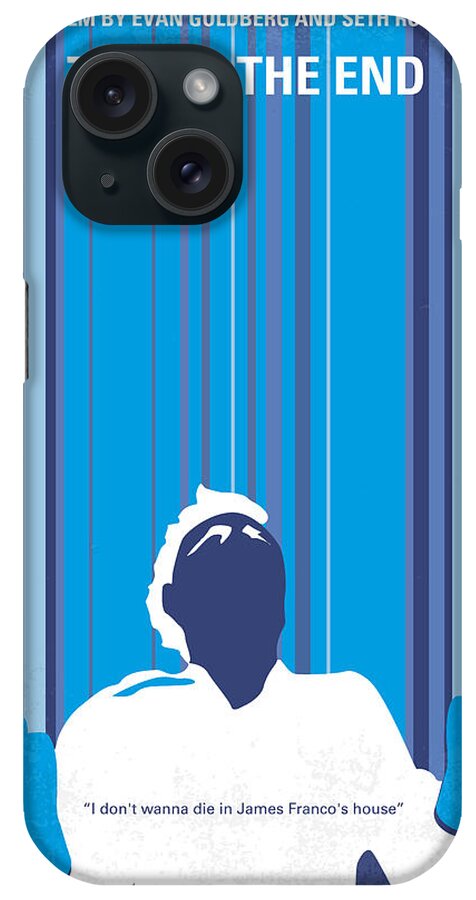This image depicts the back of a cell phone with a protective case on it, displayed against a plain white background with no visible borders. The phone, possibly an iPhone, features a rectangular shape with curved corners, measuring approximately 5 inches high and 2 inches wide. In the upper left-hand corner, there's a rounded square housing two camera lenses and a flash. Adjacent to the camera area, large white lettering states, "The End." 

At the top of the phone case, partially cut-off text reads, "by Evan Goldberg and Seth," with the rest going off-screen but likely completing as "Seth Rogan." The phone case's design includes vertical pinstripes in various shades of blue, ranging from dark navy to light blue, and purple-blue hues. 

At the bottom of the image, there is a stylized outline in white of a man reclining back on a couch. This figure has white hair, eyebrows, and a shirt, with the rest of his face in dark navy blue, lacking detailed features. Superimposed over his chest in quotations is the phrase, "I don't want to die in James Franco's house." This combination of visual and textual elements suggests a connection to the film "This Is The End," directed by Evan Goldberg and Seth Rogan.